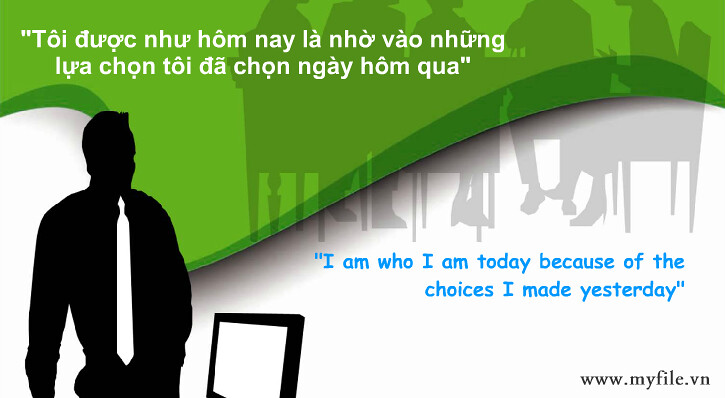This advertisement is rectangular in shape and primarily features a green and white color scheme, separated by a swirl line. At the top, there’s a green section with a quote written in Vietnamese, accompanied by another version in English on the bottom half. The English text reads, "I am who I am today because of the choices I made yesterday," followed by the website address, www.myfile.vn, in blue letters against the white background. On the left-hand side, the silhouette of a man wearing a bright white tie stands in front of a blank computer screen. In the background across the entire image, there's a black silhouette of a group of people seated around a large meeting table, evoking a boardroom or possibly a group discussion setting. The color palette includes hues of dark green, light green, white, blue, gray, and black, creating a visually striking advertisement.